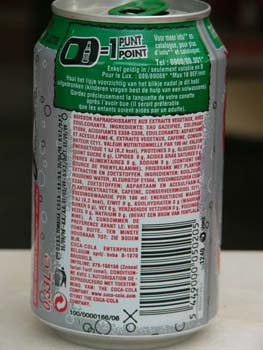This close-up image captures the back of a soda can predominantly colored in green, red, white, and silver hues. The can's primarily silver body features a green rim around the top, and the pull tab matching the rim is also green. Prominently displayed at the top of the can is black text reading "1 Punt Point," indicating that the tab can be traded for a point. Below this, the can showcases various details about its contents, including ingredients and other information, although the text is too small to decipher clearly. To the left side of the image, red text in a white rectangle includes the volume information, stating ".33 L." The barcode, positioned in the bottom right corner, is black against a white background. The can sits on a white table, with an indistinct background visible behind it.